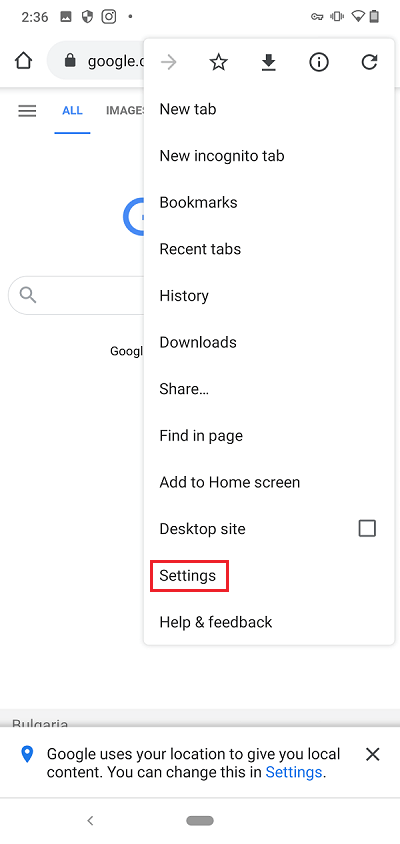This screenshot from a mobile phone displays a user actively exploring the settings on the Google website. The image captures a drop-down menu showing various options, including "New tab," "New incognito tab," "Bookmarks," "Recent tabs," "History," "Downloads," "Share," "Find in page," "Add to home screen," "Desktop site," "Settings," and "Help and feedback." Notably, the "Settings" option is highlighted with a red rectangular box, indicating the user's current focus.

At the top of the screenshot, the phone's status bar is visible, displaying the time as 2:36 and showing several icons, including a nearly depleted battery. The search bar at the top contains the word "Google," confirming the image's context.

Towards the bottom of the screen, a gray banner reads "Bulgaria," which could be either the user's location or a selected preference. Additionally, a pop-up message states, "Google uses your location to give you local content. You can change this in settings," with the word "settings" highlighted in blue. This suggests that the user is likely trying to change their location settings to access localized content.

This image offers an insightful look into how users can navigate Google settings to manage their location information effectively, ensuring they receive relevant local content.